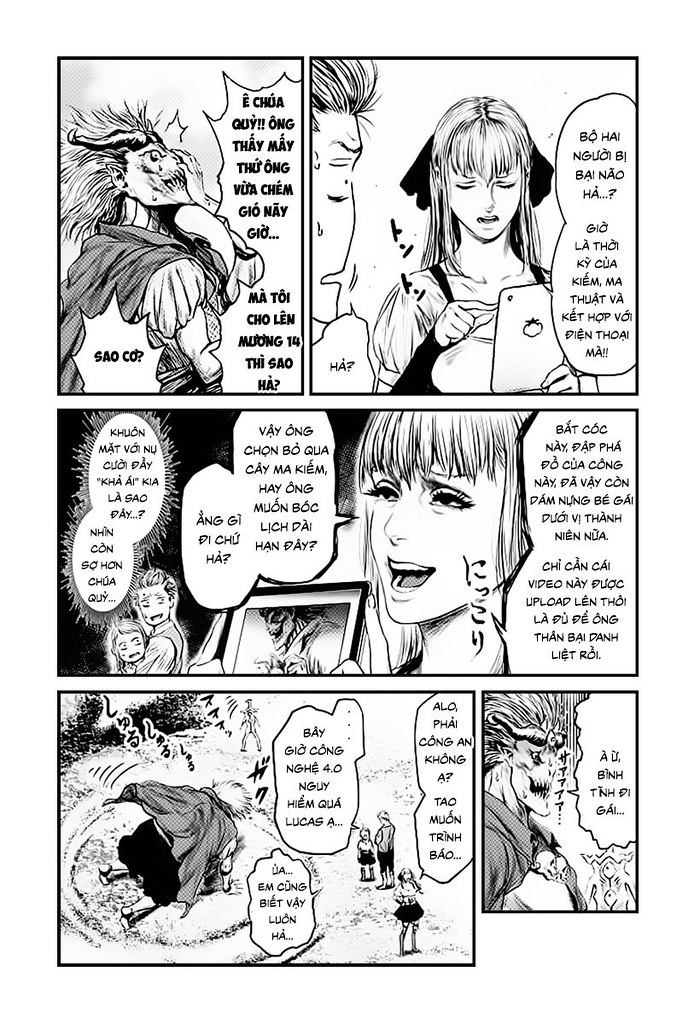This black-and-white illustration depicts a detailed comic book page in a portrait format drawn in manga-style anime, featuring several characters engaged in an intriguing scene. The comic strip, split into multiple panels, features dialogue in an unfamiliar language, possibly Asian such as Filipino or Vietnamese.

In the upper left-hand corner, a monstrous, Skeletor-like figure with horns and a cape is depicted amid a flurry of foreign conversation balloons. To his right, a young woman with a head kerchief and white blouse holds a tablet, pointing at something on its screen. Despite the ominous presence of the monster, she appears calm and focused.

The central panel captures the same young woman looking upwards, conversing as two frightened figures—a young woman and a small girl—stand behind her. Their expressions contrast sharply with her composed demeanor.

In the bottom left corner, the monster figure is seen bending forward, seemingly interacting with the environment or characters in a non-threatening manner, surrounded by more conversation balloons. Finally, the bottom right panel showcases the monster figure again, this time with a singular conversation balloon, giving the impression he is laughing.

Together, the detailed sequential art portrays a dramatic and mysterious narrative, marked by striking contrasts in character emotions and interactions.